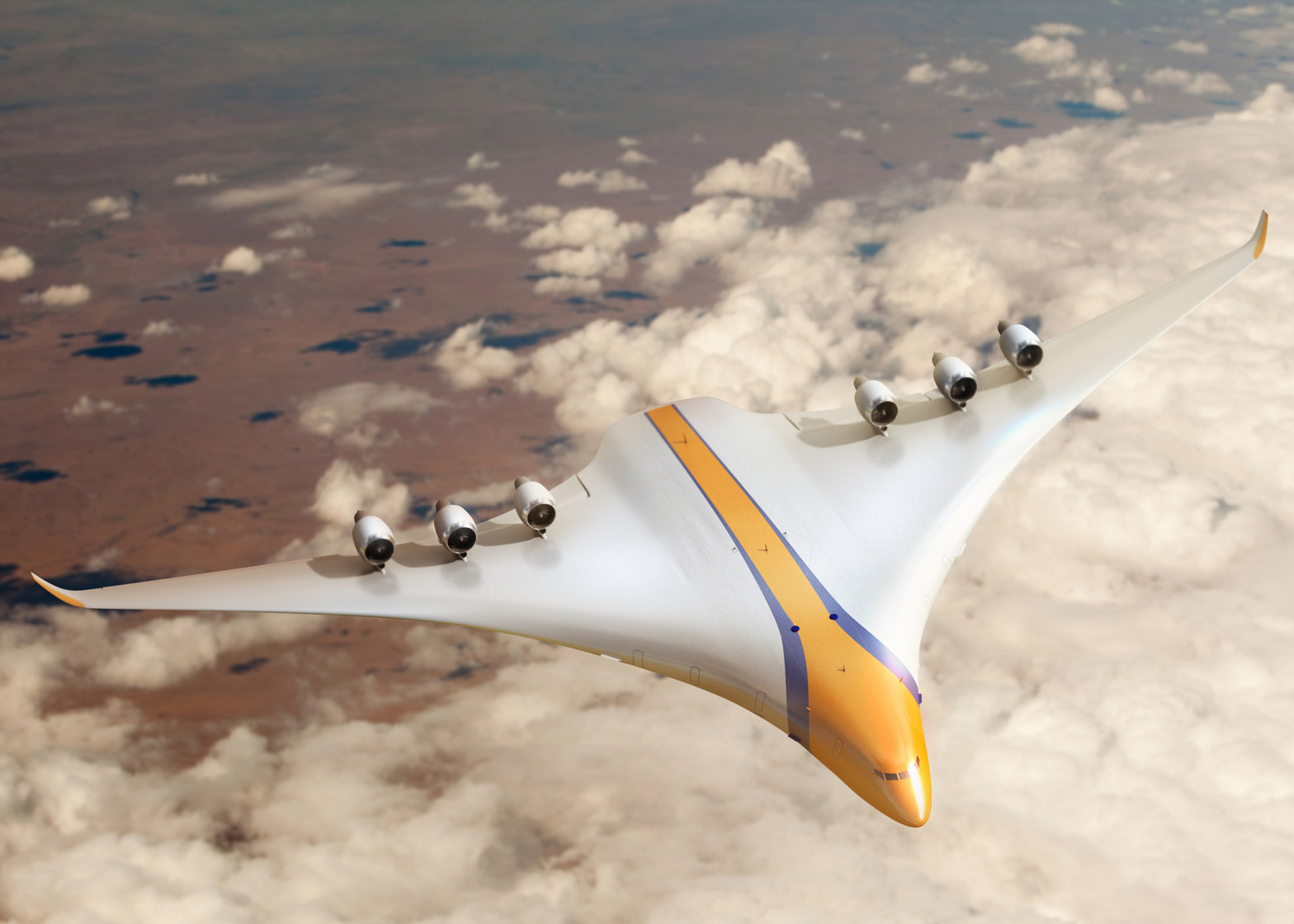The image captures a high-altitude, modernistic airplane flying over a sea of white and grey clouds, which extend across much of the background. The aircraft's unique, streamlined design features a sleek, tapered nose that elegantly curves into its wings, reminiscent of a bird in flight. The white wings, each outfitted with three jet engines, sport tips that are subtly turned upward and are accented with splashes of orange. A striking yellow stripe, embellished with thin blue trim, runs along the length of the plane's body from the cockpit to the rear. In the distant background, hints of water and islands are faintly visible, anchoring the airplane firmly in an open sky devoid of text, underscoring the image's modern and futuristic appeal.